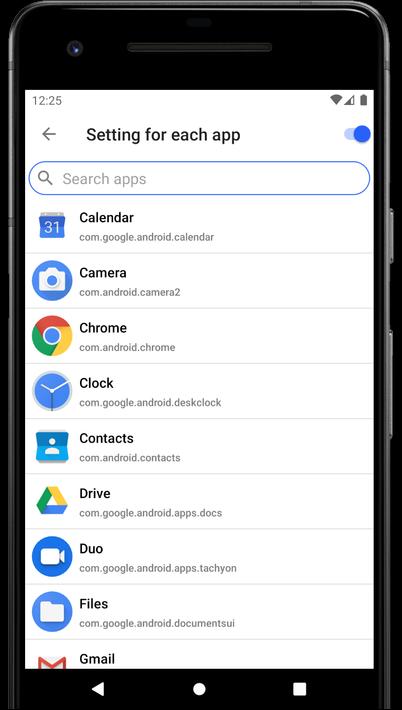A sleek black cell phone is prominently displayed against a dark background, with only its sides and buttons faintly visible due to the contrasting shadows. The phone's screen is illuminated, showcasing a white interface. In the upper left corner, the time is displayed as "12:25," while the upper right corner shows indicators for cell signal, Wi-Fi strength, and a fully charged battery.

Below these status icons, the central portion of the screen is dedicated to app settings, highlighted in blue to indicate they are toggled on. Underneath this section, there is a search bar with the placeholder text "Search apps" displayed in gray.

The screen then lists several apps in a structured format, each entry separated by a thin gray line. The apps shown include:
- Calendar (com.google.android.calendar)
- Camera (com.android.camera2)
- Chrome (com.android.chrome)
- Clock (com.google.android.deskclock)
- Contacts (com.android.contacts)
- Drive (com.google.android.apps.docs)
- Duo (com.google.android.apps.tachyon)
- Files (com.google.android.documentsui)

Every app is listed with their corresponding package names, providing a comprehensive overview of the phone's main interface layout.